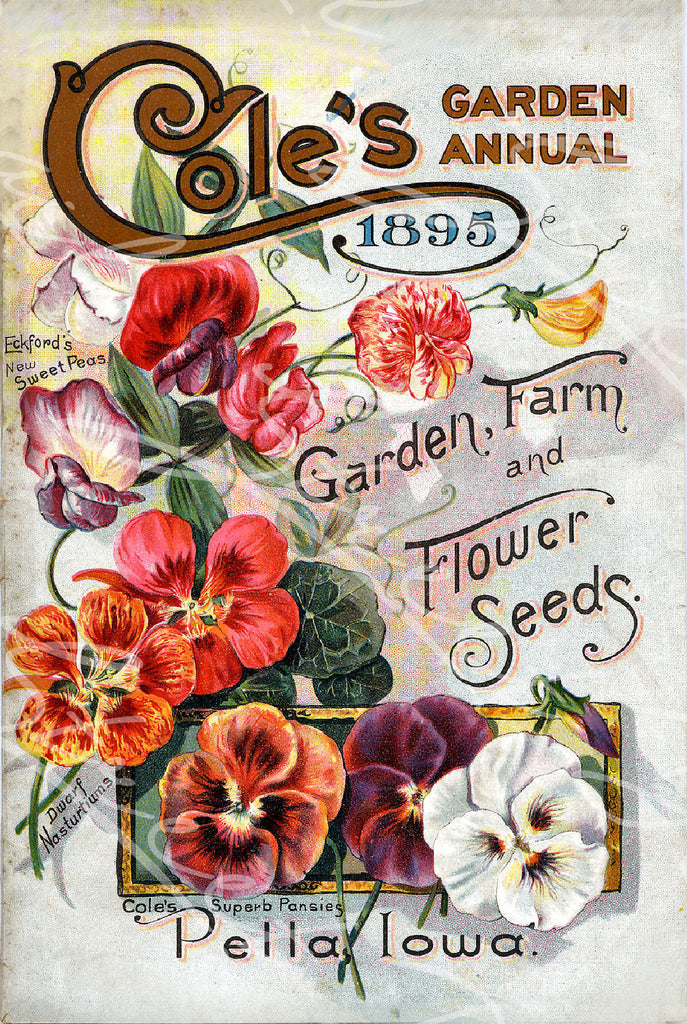This is an image of Cole's Garden Annual catalog from 1895, which serves as an advertisement for their garden, farm, and flower seeds. The cover is remarkably colorful and high-quality, especially for its time. The word "Kohl's" is written in a decorative brown font, where the capital 'C' curls around to form an oval that encloses the date "1895" in blue. Dominating the visual are vibrant illustrations of flowers. At the top, "Eckford's New Sweet Peas" is prominently displayed, showcasing an array of sweet peas in various hues, including red, purple, white, orange, and yellow. Below, "Dwarf Nasturtiums" are featured, characterized by their reddish-orange flecked petals. Further down, "Kohl's Superb Pansies" are represented by three different pansies in white, purple, and reddish-orange. The bottom of the design specifies the origin, "Pella, Iowa," emphasizing the exclusivity and high craftsmanship of the catalog in that era.